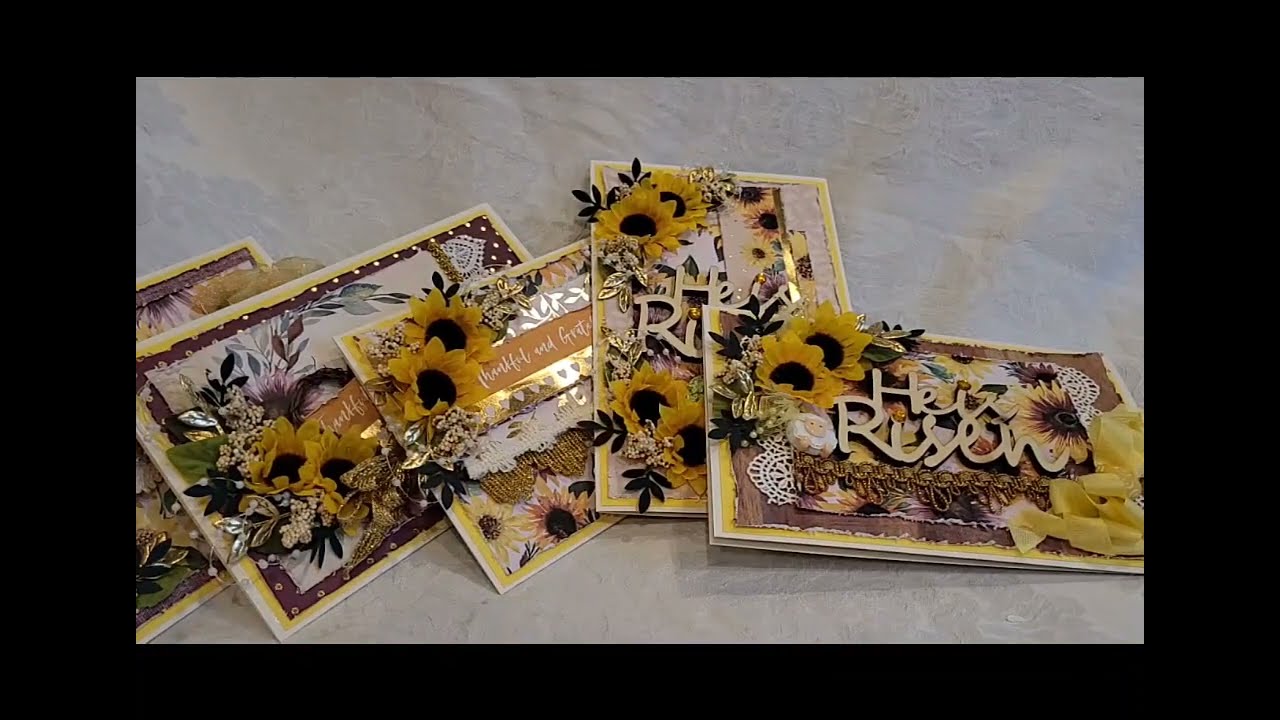The image depicts a collection of intricately designed greeting cards with a religious theme, all set against a white tablecloth background, encased by a black border. There are five cards in total, arranged with some lying horizontally, others vertically, and a few positioned diagonally. Each card prominently features yellow sunflowers with dark brown centers, complemented by yellow ribbons and white lace that lend an elegant touch. The messages on the cards include "He is risen," with some texts appearing as raised cutouts. The decorations are a mix of materials, including fabric, faux gold leaves, and shiny metallic pieces, all contributing to a cohesive color palette of yellow, white, and brown. These cards, possibly intended for church gatherings or religious celebrations, exhibit a blend of printed and glued elements, giving them a rich, textured appearance.